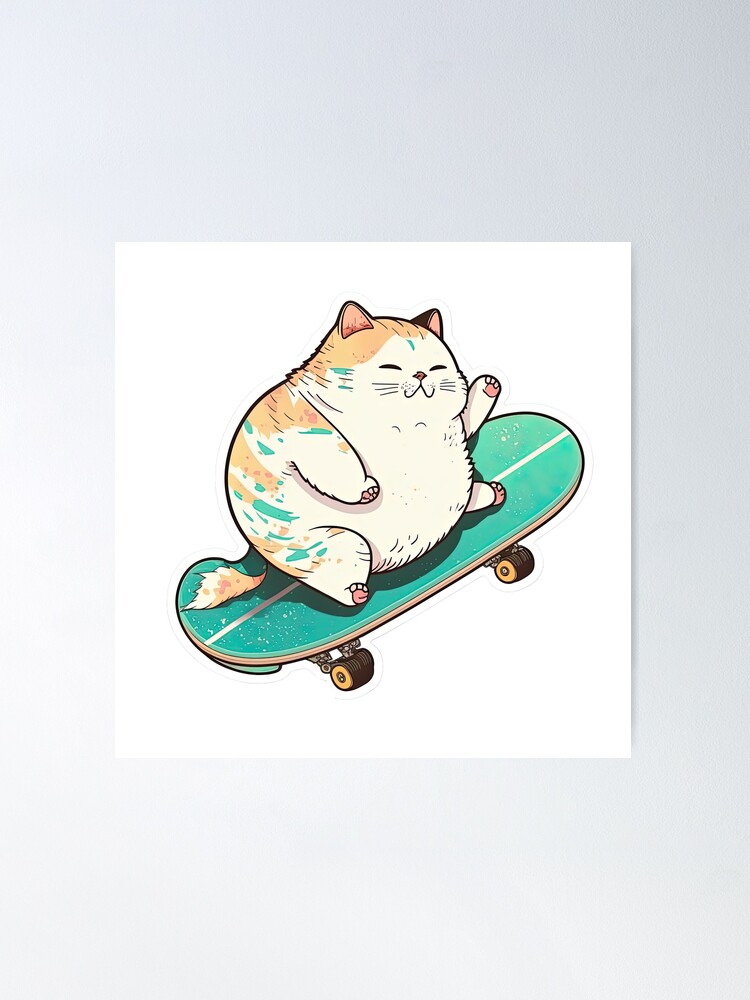The image features a cartoonish, chubby cat with a striking design, set against a gray background. This animated cat, predominantly white with orange stripes along its back and occasional green streaks, perches happily on a green skateboard adorned with a vertical white stripe. The skateboard is shown at a 45-degree angle, and features two visible brown wheels. The cat, seemingly overweight, sits with its legs spread apart, one paw raised as if waving, and a cheeky smile on its squinty-eyed face. Its tiny triangular ears peek from the top of its head, colored pink inside. The detailed black outline accentuates the cat's rotund form, which lacks a clear neck, enhancing its tubby appearance. The entire scene appears to be depicted on a white poster, adding a minimalist contrast to the playful and vibrant subject.